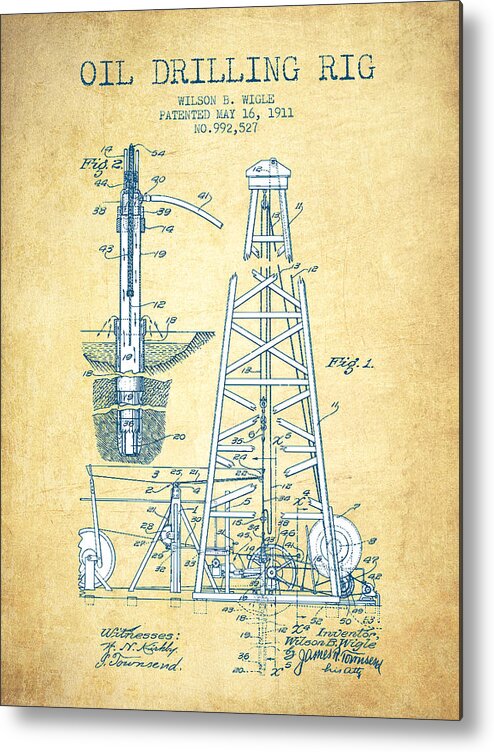This schematic drawing, presented on a vertically elongated, dingy beige paper typical of early 20th-century documents, displays an oil drilling rig titled "Oil Drilling Rig" in green text. Underneath, it reads "Wilson B. Wiggle, Patented May 16, 1911, No. 992,527." The document, likely a patent illustration enlarged for display, features detailed diagrams of the oil rig. On the right side, "FIG 1" showcases the overall structure of the rig, including a tower adorned with numerous mechanical components, each meticulously numbered. The left side provides a closer look at the interior mechanics, potentially focusing on the drill part. Both diagrams, labeled with arrows pointing to various parts, show different aspects of the rig, one emphasizing its drilling depth. Additional handwritten names at the bottom include inventors Wilson B. Wiggle and a partially legible James B. Townsend, witnesses H.N. Kirby and J. Townsend, adding a historical, personal touch to the technical rendering.